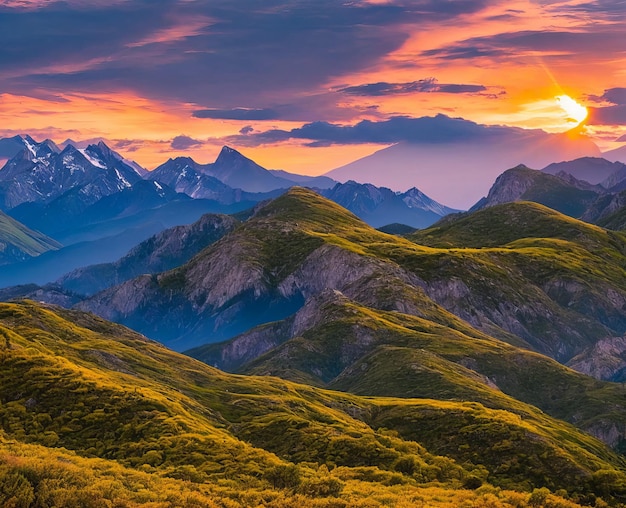This captivating photograph captures a breathtaking mountainscape at either sunrise or sunset. The foreground showcases a series of rolling mountains adorned with lush greenery and tall grasses, all devoid of trees or human presence. The mountains further back on the left are partially bare and dotted with snow, indicative of a higher elevation. Another distant mountain range can be discerned on the far right. The sky is a brilliant tapestry of oranges, yellows, pinks, and purples, illuminated by the rising or setting sun emerging from behind a cluster of clouds. This dramatic lighting casts a mystical hue over the scene, accentuated by streaks of mist or fog threading through the valleys. The overall composition captures the serene, untouched beauty of the mountainous landscape.